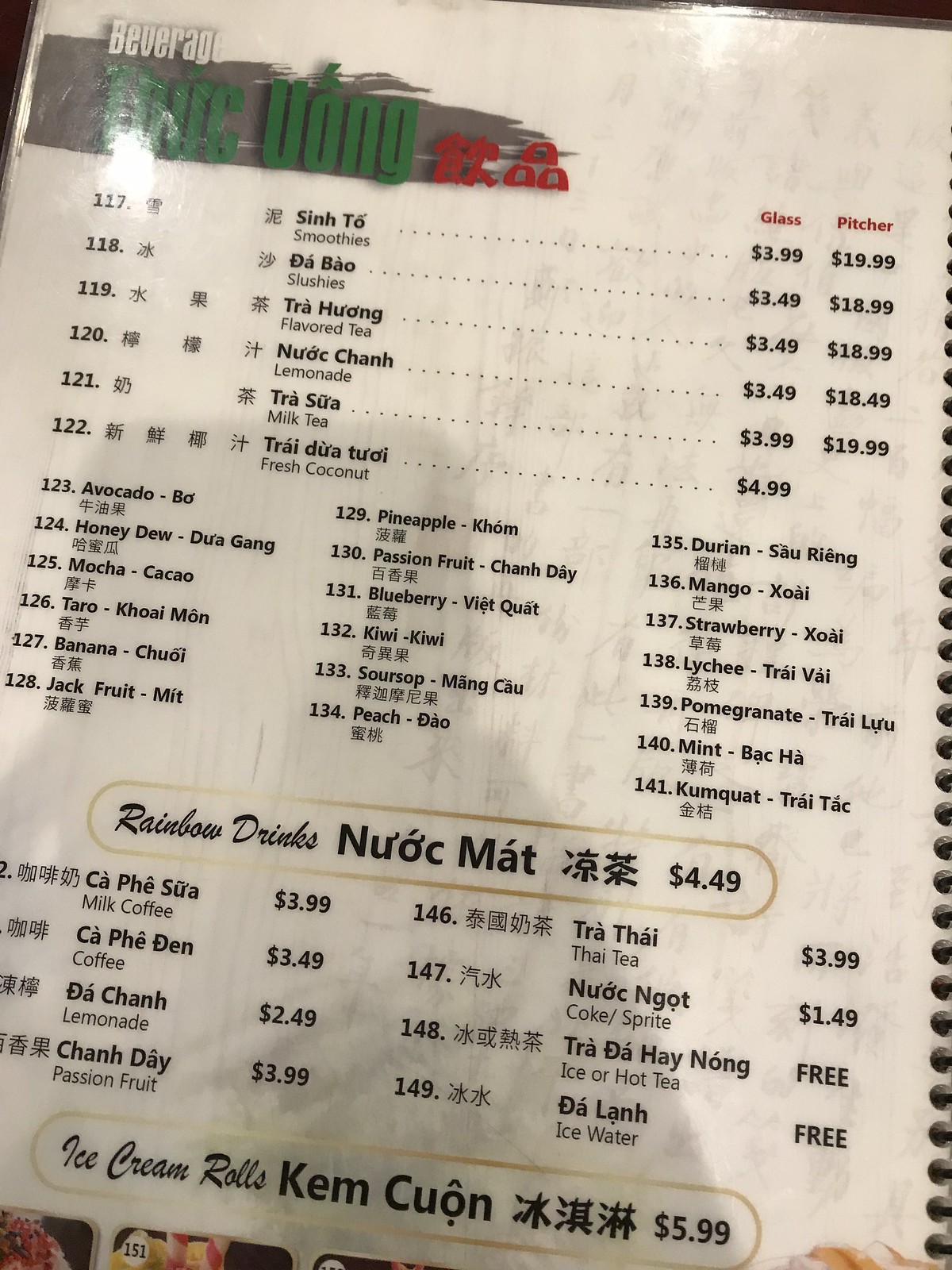Photograph of a restaurant menu. The menu is encased in a black binder with metal loops binding the pages, giving it a sturdy and organized appearance. The background of the menu is a clean white color. 

In the upper right-hand corner, the heading "Beverages" is prominently displayed, followed by "Thick Yong" and some Japanese or Chinese characters.

The menu is detailed as follows:

- **117. Sinto Smoothies**: $3.99 for a glass, $19.99 for a pitcher.
- **118. Dabao Slushies**: $3.49 for a glass, $18.99 for a pitcher.
- **119. Trae Hyung Flavored Tea**: $3.49 for a glass, $18.99 for a pitcher.
- **120. New York Chan Lemonade**: $3.49 for a glass, $18.49 for a pitcher.
- **121. Trae Sua Milk Tea**: $3.99 for a glass, $19.99 for a pitcher.
- **122. Trae Dua Tou Fresh Coconut**: $4.99.

Following these are individual items listed with fruit or flavor names:

- **123. Avocado**
- **124. Honeydew**
- **125. Mocha**
- **126. Taro**
- **127. Banana**
- **128. Jackfruit**
- **129. Pineapple**
- **130. Passion Fruit Chande**
- **131. Blueberry Viet Quat**
- **132. Kiwi Kiwi**
- **133. Sour Soup Ming Kao**
- **134. Peach Dao**
- **135. Durian San Reng**
- **136. Mango Jiao**
- **137. Strawberry Jiao**
- **138. Leche Trae Viao**
- **139. Pomegranate Trae Lu**
- **140. Mint**
- **141. Kam Quat Trae Tak**

Additionally, the menu features:

- **Rainbow Drinks Kyok Matt**: $4.49, with flavors such as Milk, Coffee, Lemonade, Passion Fruit, Thai Tea, Coke, Sprite, Ice or Hot Tea, or Ice Water.
- **Ice Cream Rolls Kim Kyon**: $5.99.

The menu is comprehensive, providing a wide array of beverage options, from smoothies and teas to slushies and refreshing fruit drinks, as well as unique ice cream rolls.